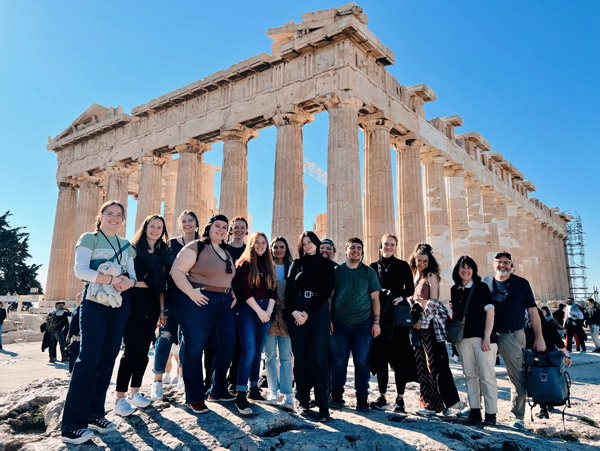This image captures a group of approximately 20 people, a mix of males and females, posing in front of the ancient ruins of what appears to be the Parthenon in Greece. In the center of the group, likely consisting of high school or college-aged students on a school trip, two adults—presumably teachers—stand to the right. The ruins, featuring tall stone columns and a partially intact structure with no roof, stand prominently in the background, their brown and white stone showcasing the wear of time. The group is arranged on rocky ground, with some members holding backpacks and perhaps even a baby or two. The background also includes other tourists examining the historical site, while the clear blue sky with no visible clouds suggests it is a bright, sunny morning. Trees frame the left side of the image, adding a touch of greenery to the ancient scenery.